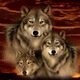The image is very small, about the size of a thumb, and square in shape. It depicts three wolves positioned centrally against a backdrop that gives a red, cloudy impression, resembling a brick wall. The largest wolf is situated above the other two, while the medium-sized wolf is to the left of the smallest one. All three wolves have typical gray, white, and light brown hues. The two larger wolves are looking directly at the camera, while the smallest wolf gazes towards the bottom left corner. The background transitions from red clouds to a black lower section, enhancing the distinct, intense gaze of the wolves. The overall setup almost suggests a family grouping, with detailed facial features and fur colors clearly visible despite the image's small size.